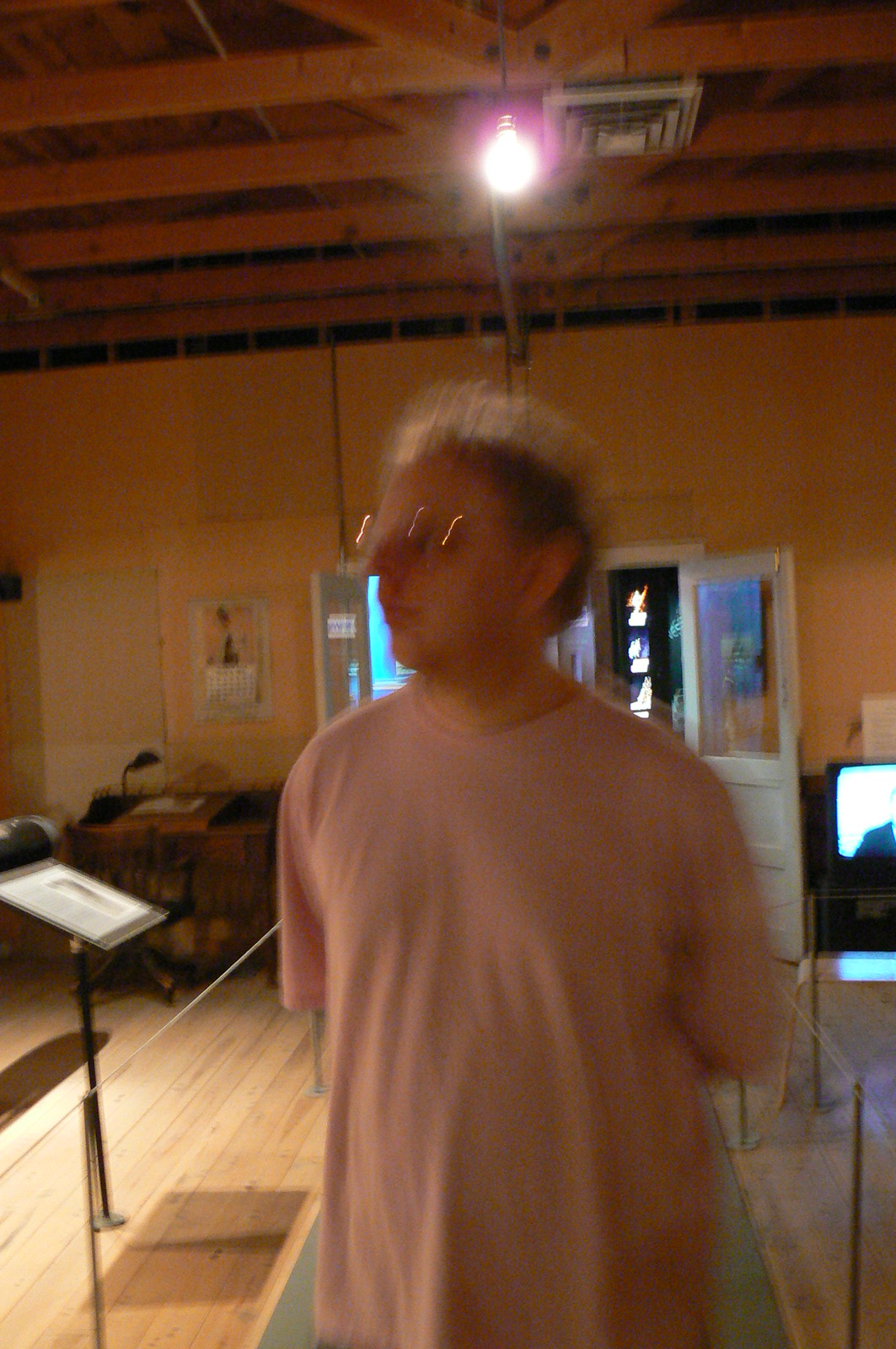In this rectangular, low-resolution photograph taken inside a room, we see a blurry close-up of a man positioned at the center of the image. He is wearing an oversized peach-colored t-shirt that covers him from the lower waist up, with only the t-shirt's sleeves visible at his sides. His arms appear to be bent at the elbows and positioned behind him. Although his facial features are difficult to discern due to the blurriness, the light reflecting off his glasses is noticeable. He has fair-colored, medium-length hair that reaches the base of his neck, and he is gazing towards the west while his body faces forward.

The setting seems to be a classroom, discernible by the double white doors behind him and a podium situated to the west side of the image, which has a white piece of paper placed on it. There’s also a desk in the far left corner of the room. The classroom features a wooden floor and what appears to be a screen in the upper right corner.